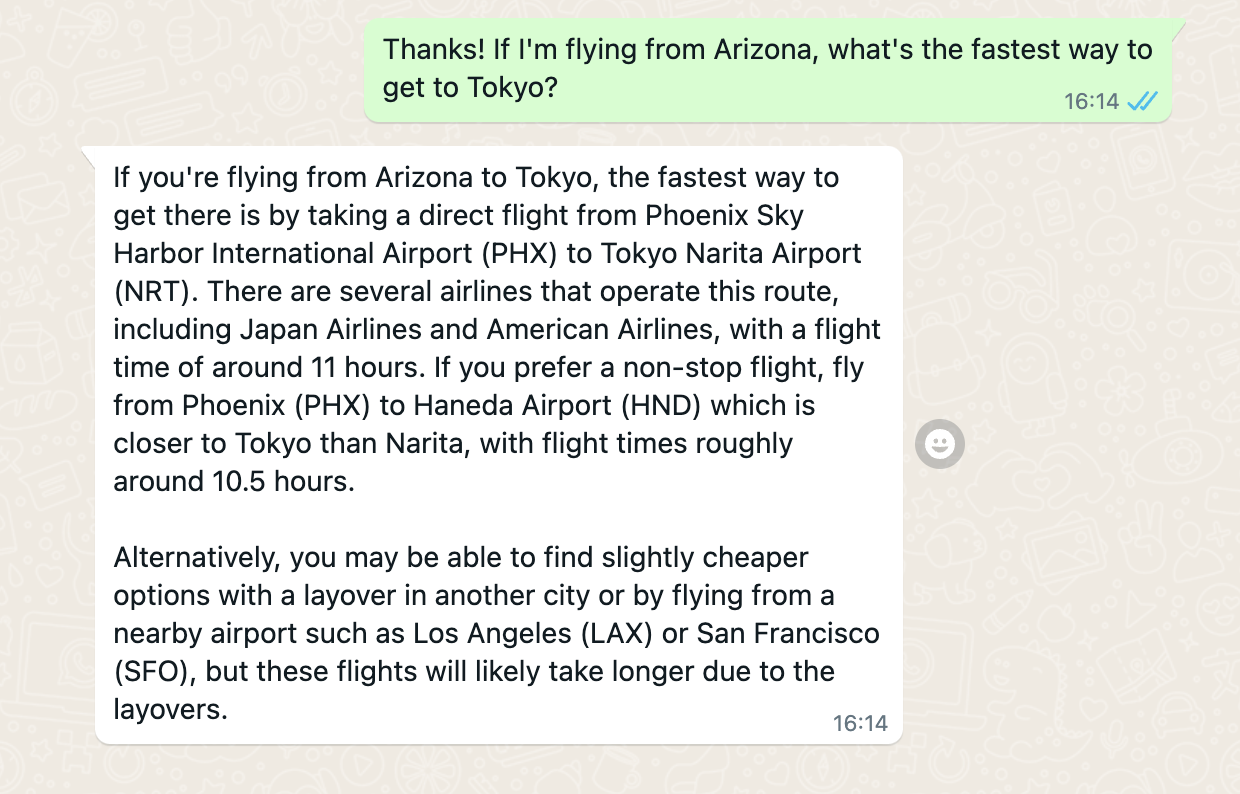The image is a screenshot of a conversation between two people on a messaging platform. At the top right, there's a green chat bubble with black text that reads, "Thanks, if I'm flying from Arizona, what's the fastest way to get to Tokyo?" This message is timestamped at 16:14. Below it, in a larger white chat bubble with black text, the response reads: "If you're flying from Arizona to Tokyo, the fastest way to get there is by taking a direct flight from Phoenix Sky Harbor International Airport to Tokyo Narita Airport. There are several airlines that operate this route, including Japan Airlines and American Airlines, with a flight time of around 11 hours. If you prefer a non-stop flight, fly from Phoenix to Narita Airport, which is closer to Tokyo than Narita, with flight times roughly around 10 and a half hours. Alternatively, you may be able to find slightly cheaper options with a layover in another city or by flying from a nearby airport, such as Los Angeles or San Francisco, but these flights will likely take longer due to the layovers." The background of the image is a subtle, slightly tannish off-white with delicate white designs.